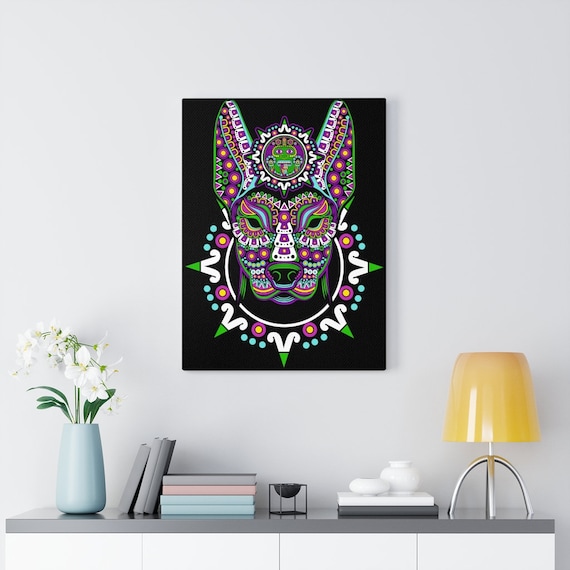This photograph captures a tastefully decorated interior scene featuring a sleek gray and white desk with a dark gray top. Positioned on the right side of the desk is a striking yellow lamp. On the desk's surface, there are several ceramic pieces, possibly vases, interspersed among a collection of pastel and gray books that include shades of pink and blue. To the left, a potted plant with white flowers sits elegantly in a light blue vase. Above this arrangement, a plain white wall showcases an eye-catching abstract piece of artwork. The painting, with a black background, depicts a dog's face composed of various colorful shapes and designs. The multicolored dog features notable details like purple circles with yellow centers, purple triangles, and intertwined hues of green, orange, and blue. The dog's head is encircled by an orb featuring additional abstract facial elements, including small round dots and a sharp, pointed V shape. This eclectic framed artwork attracts attention with its vibrant use of colors and geometric patterns, adding a dynamic focal point to the otherwise minimalist space.